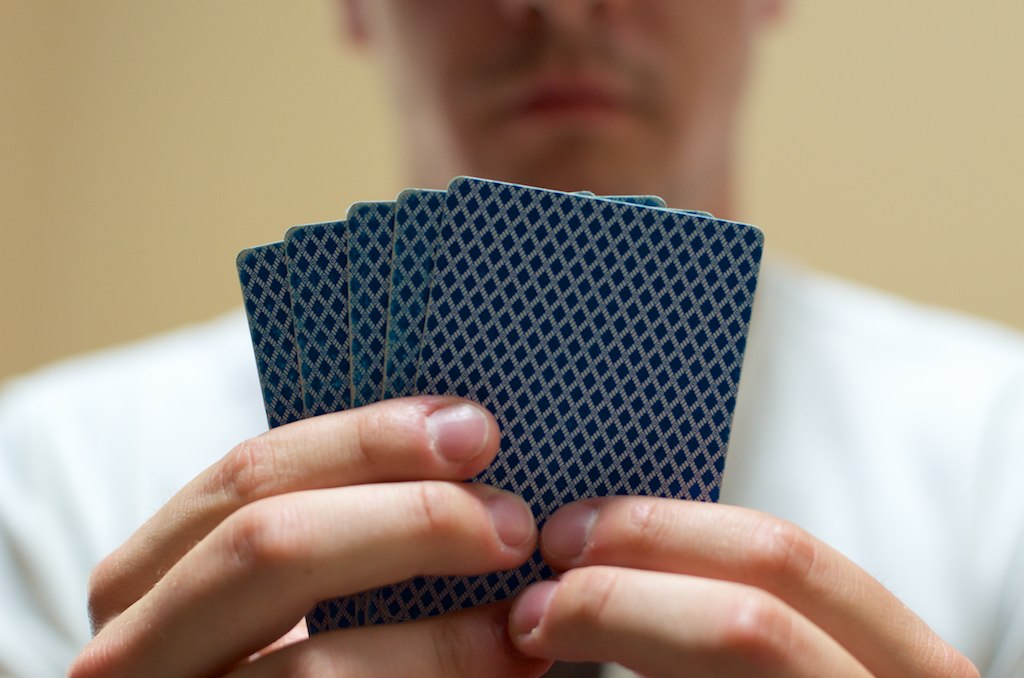A close-up stock photograph captures a male Caucasian, identified by his visible clean fingernails and white shirt, sitting across from the viewer. The focus of the image is on his hands, which tightly grasp five fanned-out playing cards featuring a blue, diagonal cross-hatching pattern with white stripes on their backs. The scene is set against a tan background. The man's face and upper torso are intentionally blurred and partially cut off above the nose, emphasizing the playing cards and his decision-making process. The tight crop on the hands and cards suggests a strategic moment in gameplay.